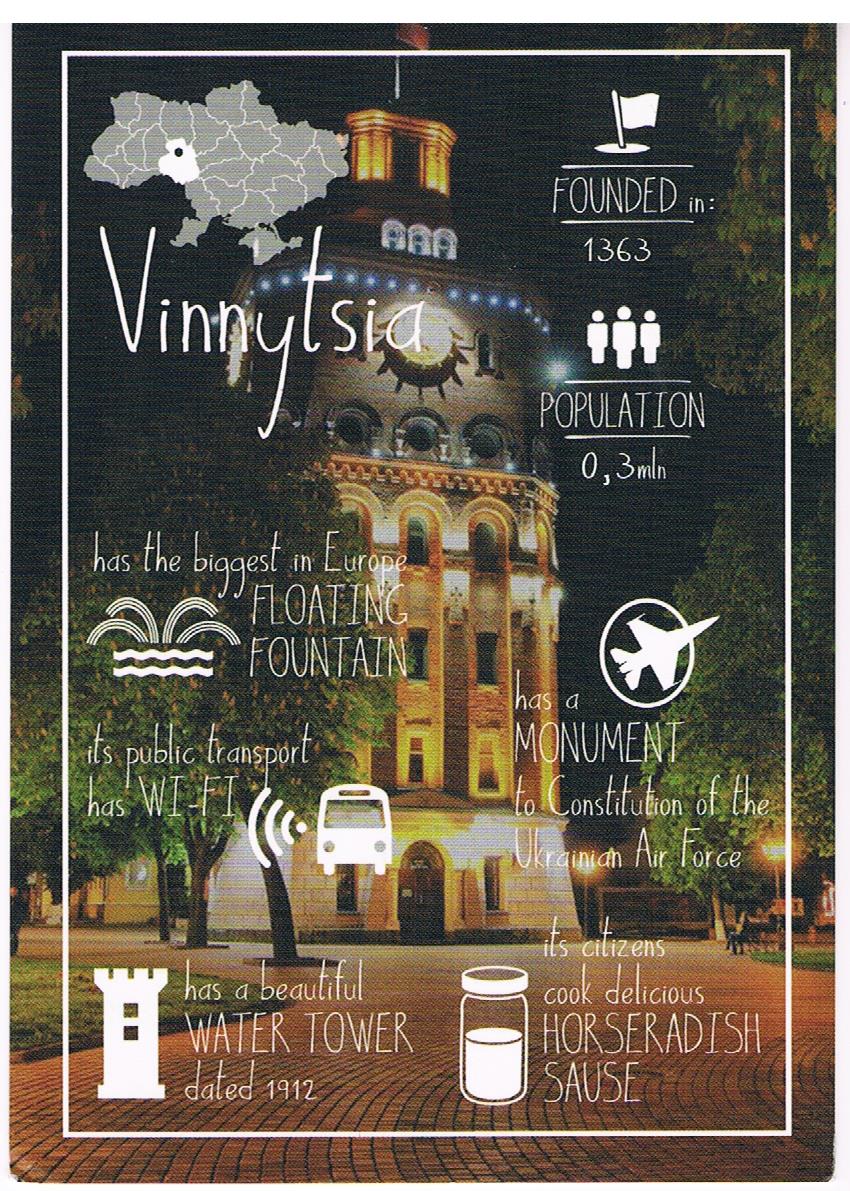The image displays a slightly distorted, printed travel poster with a nighttime photograph of a well-lit tower, accompanied by a neatly landscaped brick pathway, grass, and trees. The poster advertises Venetia (spelled "V-I-N-N-Y-T-C-T-S-I-A"), a city founded in 1363 with a population of 0.3 million. It highlights several key attractions: Europe’s largest floating fountain, a monument to the Constitution of the Ukrainian Air Force marked by a logo of a fighter jet, and a beautiful water tower dating back to 1912, symbolized by a castle-like icon. The poster also mentions the city's public transport system equipped with Wi-Fi, as indicated by a bus and Wi-Fi signal icon. Additionally, it notes that Venetia's citizens are known for cooking delicious horseradish sauce, represented by a jar icon. A map showing the city's location on its continent with a highlighted area and black dot is included. The scene is colorful, featuring a tall, 7-8 story building with blue and yellow lights, and green trees flanking the tower, blending historical and modern elements under a night sky.